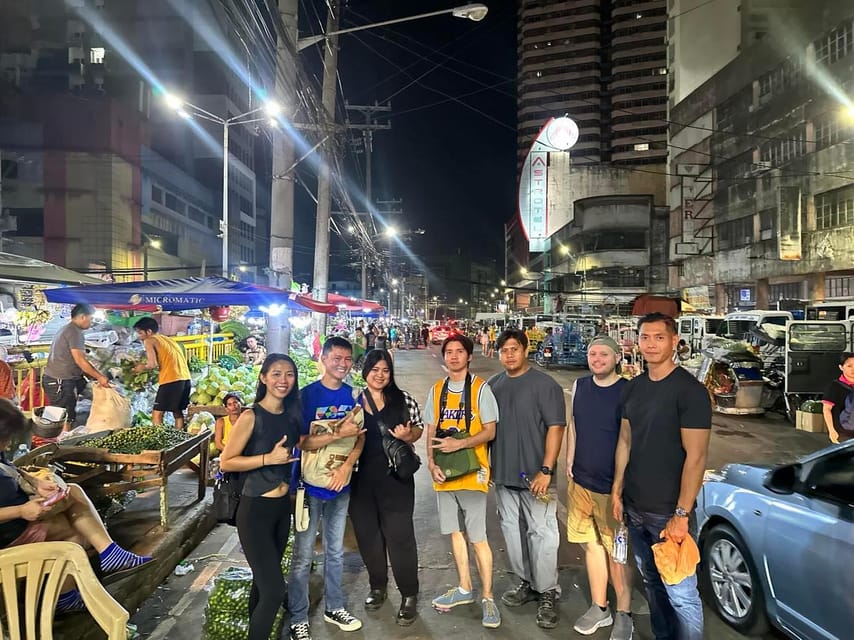In this night-time city street scene, a group of seven people—two women and five men—stand at the center, posing and smiling for the camera. Their casual attire hints at a relaxed gathering at a bustling street market. They stand beside a blue or silver sedan, with dim lit lampposts and worn-down buildings in the backdrop. The market is lively, with people shopping for produce; green, round vegetables can be seen on the left as a man in a yellow shirt fills a bag held by another. Some of the group are making hand gestures, while the rest have expressions ranging from smiles to neutral, creating a dynamic focal point amidst the vibrant, busy scene. The black sky looms overhead, void of stars or the moon, enhancing the urban night ambiance.